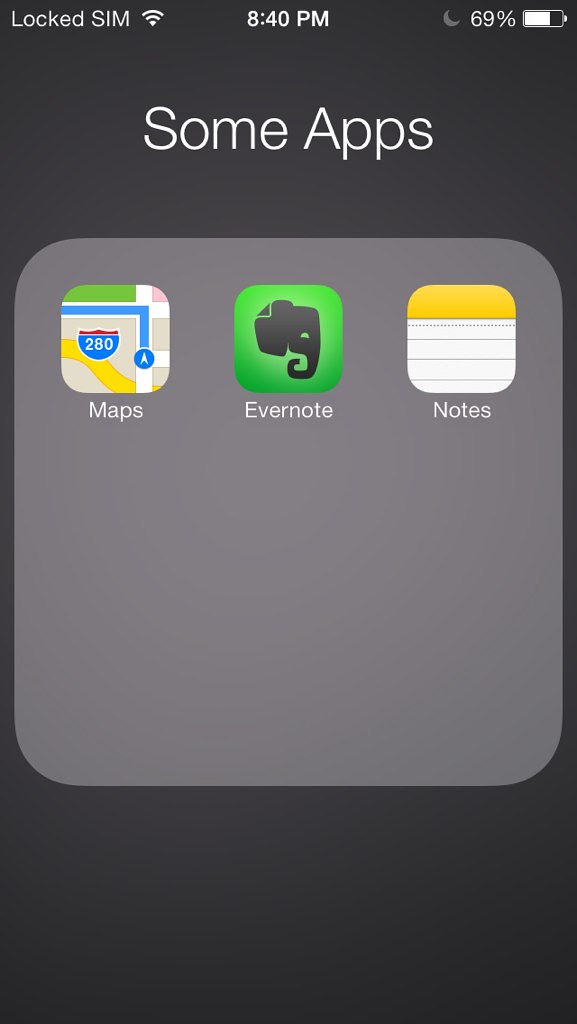Screenshot Description:

The image is a screenshot of a smartphone with a minimalistic black background. At the top of the screen, the status bar displays "Lock Sim," indicating that the SIM card is locked. Accompanying this, the status bar also shows a strong network signal, the current time (8:40 p.m.), and the battery life (69%).

At the center of the screen, there is a folder labeled "Some Apps," which contains three applications. The folder has a light gray square border, sharply contrasting the dark charcoal gray background of the device. 

The first app in the folder is "Maps," featuring a visual snippet of Interstate 280 with a few surrounding streets. The second app is "Evernote," identifiable by its distinctive black elephant logo set against a green background. The third app is a generic note-taking application, represented by an icon resembling the top view of a legal pad, featuring a yellow binding strap and lined paper beneath it.

Overall, the screenshot highlights the phone's user interface with a clear and organized display of apps against a simple yet sleek dark background.